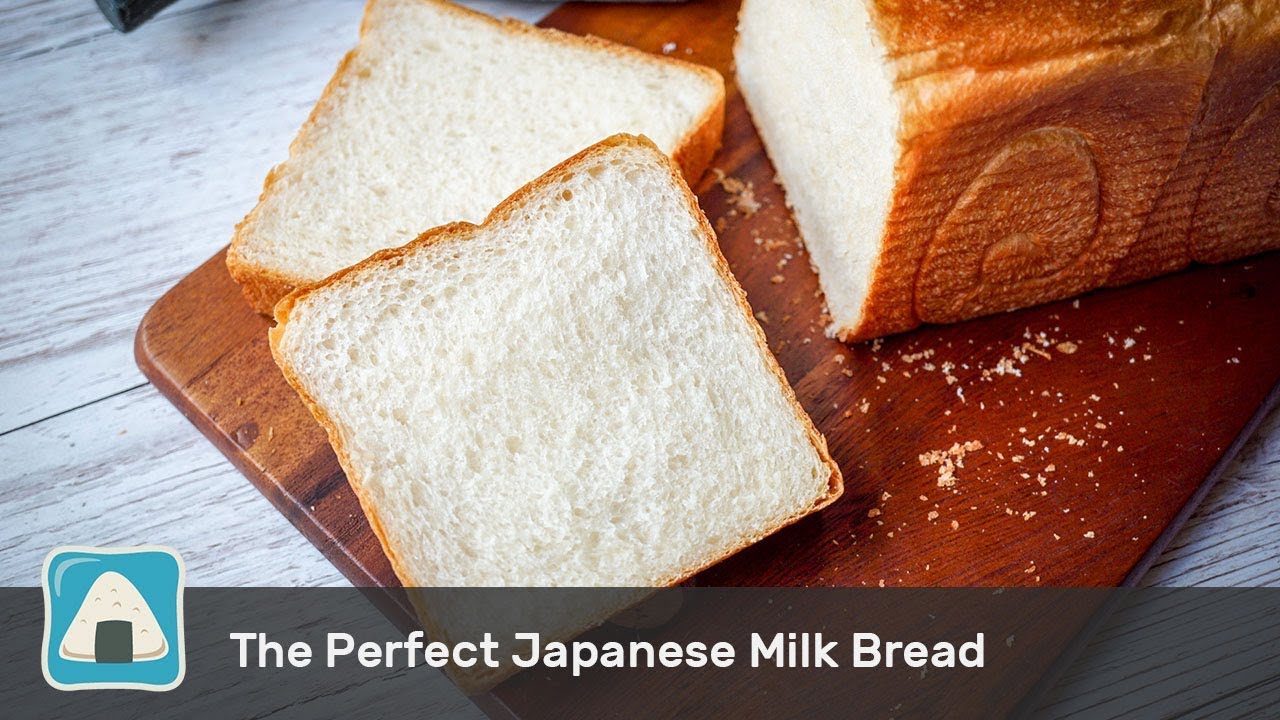The image showcases a freshly baked loaf of bread, artfully placed on a dark brown wooden cutting board. The cutting board rests on a diagonally grained grayish-silver table, adding a subtle but striking contrast. Positioned in the upper right of the frame, the bread loaf is adorned with intricate swirly designs and horizontal lines. Two neatly sliced pieces of bread, white with brown crusts, lie partially overlapping to the left of the loaf, amidst a few scattered crumbs. At the bottom of the image, a gray banner runs horizontally, featuring an icon resembling a piece of bread with a blue background and a white triangular center. Adjacent to this icon, bold white lettering declares, "The perfect Japanese milk bread."